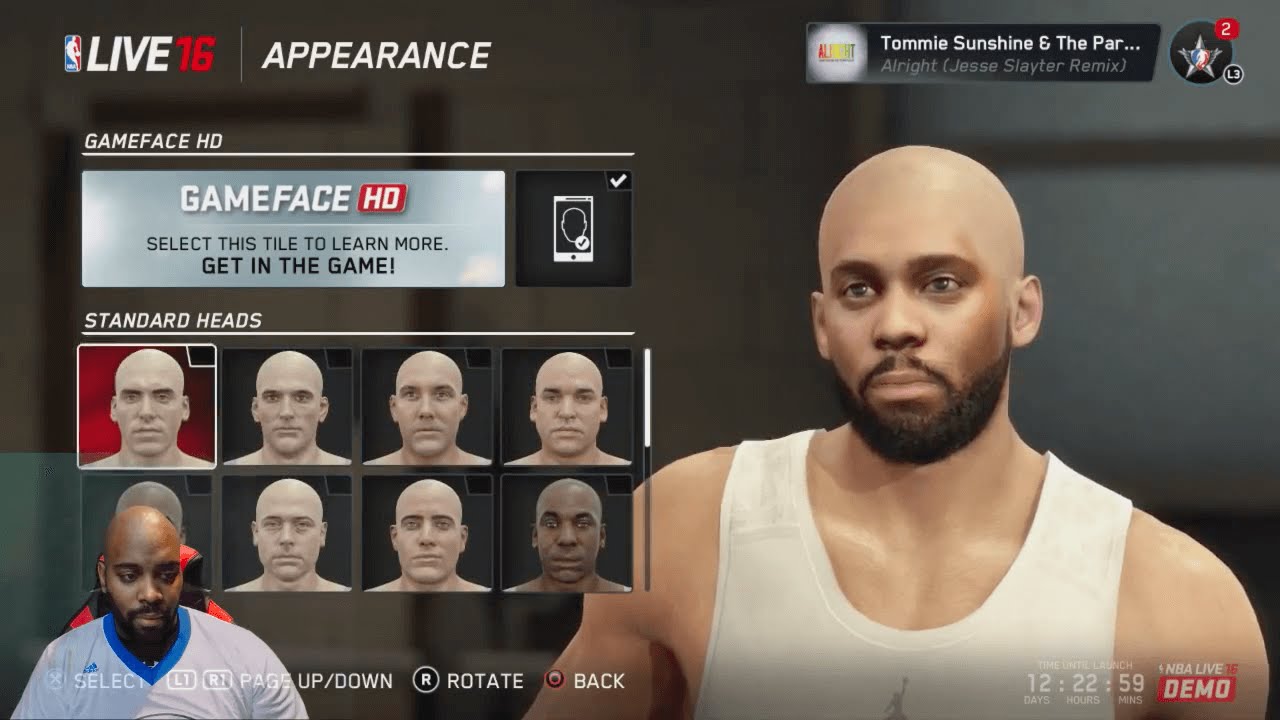This image is a detailed screenshot of a live stream featuring a gamer customizing an avatar in the game NBA Live 16. In the bottom left corner, the streamer, a bald black man with a black beard and mustache, is visible. He is wearing a white jersey with a blue collar. 

The main screen showcases the "Appearance Selection" section. At the top, the text "LIVE 16" is prominently displayed, with 'LIVE' in white and '16' in red, accompanied by the NBA logo on the left. Below this, there are options titled "Appearance" and "Game Face HD." The "Game Face HD" option is highlighted in a gray box with the prompt, "Select this tile to learn more, get in the game."

Below these options, there are two rows of four standard head selections, each differing in facial features like jaw, nose, and mouth. In the top right corner of the screen, the music track "Tommy Sunshine and the PAR..." (Jesse Slater Remix) is indicated as playing. Additionally, there are two notifications visible next to the music information.

The streamer’s avatar, seen in the game, is a muscular, bald black gentleman with a beard, mirroring the streamer's real-life appearance. He is also adorned in a white jersey. At the bottom of the screen, various controls such as "Back," "Page Up and Down," "Rotate," and "Back" are visible, along with a countdown for an NBA Live demo.

This detailed scene effectively captures the nuances of the live streaming setup and the customization interface in NBA Live 16.